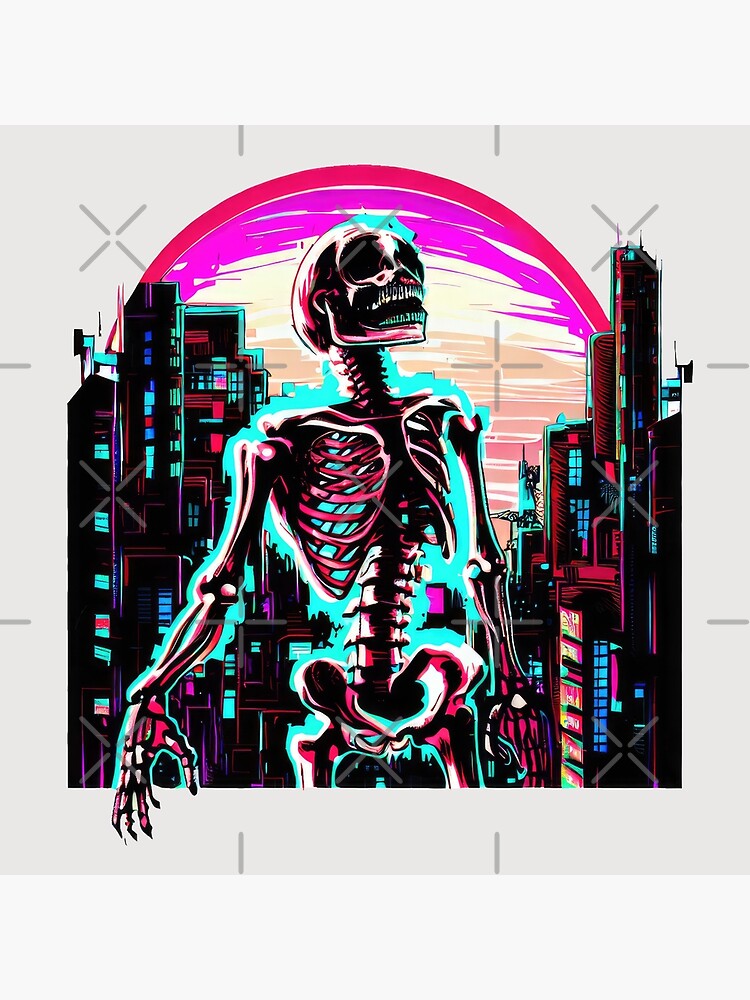In this vibrant and detailed artwork, a large, neon-colored skeleton stands prominently against a cyberpunk cityscape. The background features a light gray base with small, cross-like patterns and a mystical sky bathed in purples and pinks with a striking pink sun. Tall, high-rise buildings, predominantly black, are adorned with turquoise, green, and blue outlines, shimmering with colorful windows and accents, including some red signs.

The skeleton itself is a centerpiece of vivid neon hues. Its bones are outlined in various colors, such as turquoise, green, pink, red, and purple, and its ribs, backbone, and pelvis are intricately detailed. A blue border uniquely frames the entire skeleton, enhancing its aesthetic appeal against the bustling city. The overall composition presents a blend of comical and surreal elements, creating a lively and dynamic scene.